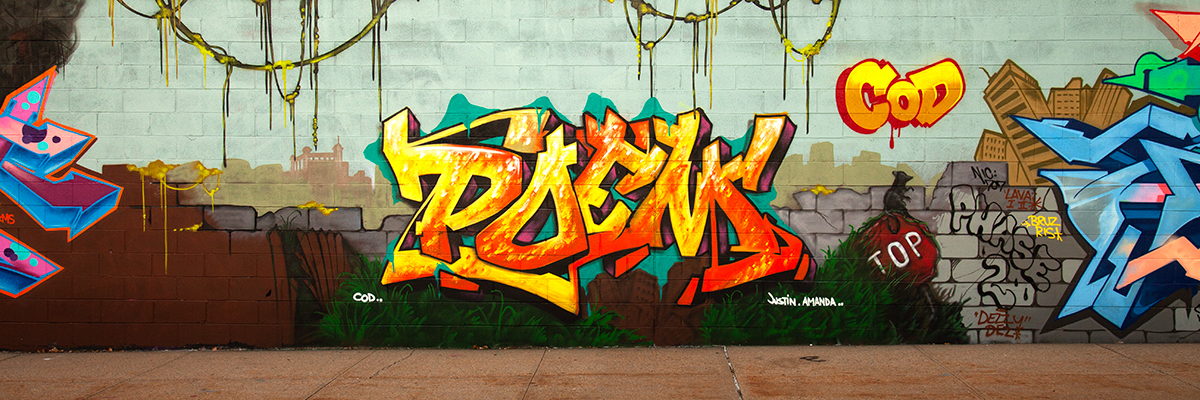This is a high-quality, panoramic color photograph of a detailed graffiti wall, vibrant with neon, cartoony artwork. The wall, made of either brick or cement, is completely covered in various graffiti sections. In the center, the word "POEMS" is prominently written in a bold graffiti style, featuring yellow, orange, and red letters. To the right of this, in similar yellow and orange hues, is the word "COD," and beneath it is a red bomb design with the acronym "TOP" in white lettering. Additionally, there is a partially hidden stop sign showing only "T.O.P." Below the main text, there's another graffiti element reading "phase two" in bubble text. The left side of the wall is adorned with more graffiti, characterized by neon pink and blue, while the right side features gray and blue artwork. At the top of the image, graffitied vines hang down, adding to the intricate details of the scene. The bottom of the wall includes a light brown tile patch, contrasting with the vivid neon colors above. The scene is completed with additional graffiti depicting buildings toppling over, enhancing the chaotic, urban aesthetic.